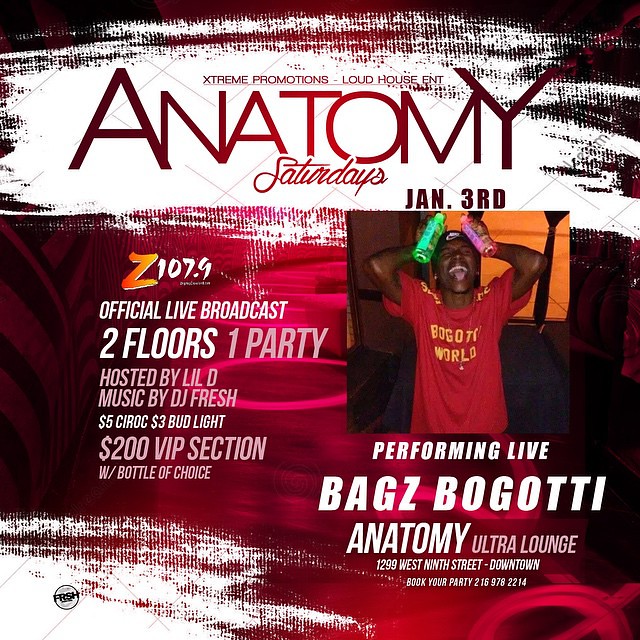The image is an advertisement flyer for a music event organized by Extreme Promotions and Loud House Entertainment. The background features a bold red graphic design. At the top, in striking red text, it reads "Extreme Promotions Loud House ENT." Below that, in large crimson red letters, is "ANATOMY," followed by "Saturdays" in cursive.

On the right side of the flyer is a vibrant image of an African-American man with stud earrings. He is wearing a backward black Nike baseball cap and a red short-sleeve T-shirt that says "Bagot World" in yellow letters. The man has his eyes closed and his tongue sticking out, and he holds a green bottle in one hand and a pink bottle in the other, pressing them against each side of his head.

To the right of this image, it notes the date "January 3rd" and "Z 107.9 Official Live Broadcast." Below this, it reads "Two Floors One Party," "Hosted by Little D," and "Music by DJ Fresh." Additionally, the flyer mentions special offers such as "$5 Ciroc," "$3 Bud Light," and a "200-hour VIP section with a bottle of choice."

At the bottom in white text, it states, "Performing Live Bags Bogatti Anatomy Ultra Lounge." The overall design merges red and black elements, creating a striking and energetic promotional piece.